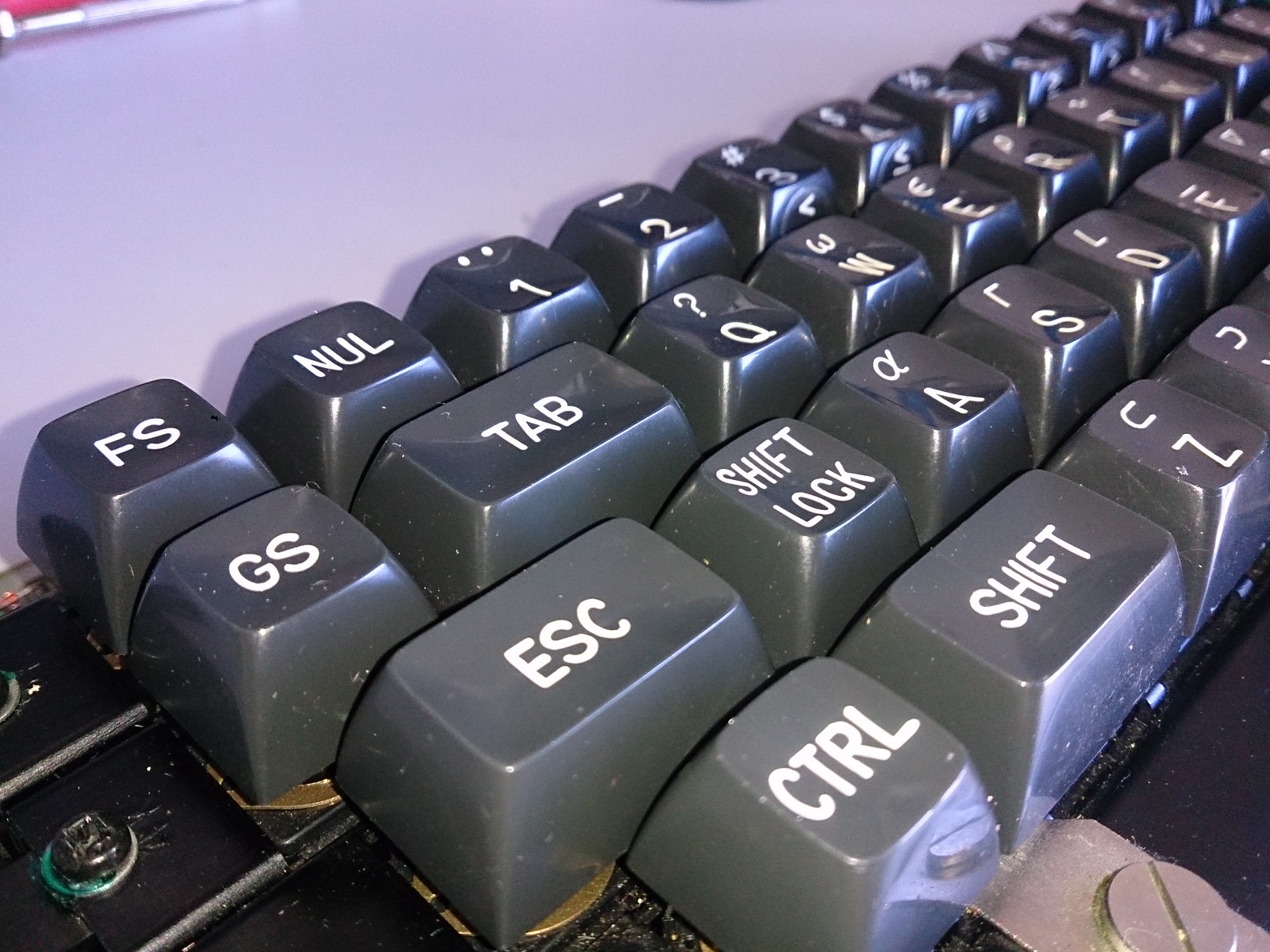A close-up, three-quarters view color photograph of an old, gray keyboard with white uppercase letters, arranged in a QWERTY layout. The keyboard appears to be bolted to a black or possibly military-green base, and its left side occupies the lower left corner of the image, while the right side extends to the top right corner. The keyboard's shadow is cast on a white background due to a light source on the right. The keys are thick and arranged diagonally, with some showing non-standard symbols like "FS," "GS," and "NULL," alongside typical keys like "CTRL," "SHIFT," and "ESC." Several screws and brass washers can be seen securing the keyboard, adding to its rugged, vintage look. The photograph, possibly of a typewriter or an ancient computing device, also shows hints of a lighter-colored object and a small red or pink sliver in the background, with some golden twine or wire visible underneath the keys. The overall appearance is somewhat dirty, suggesting the keyboard is outdated and in need of cleaning.